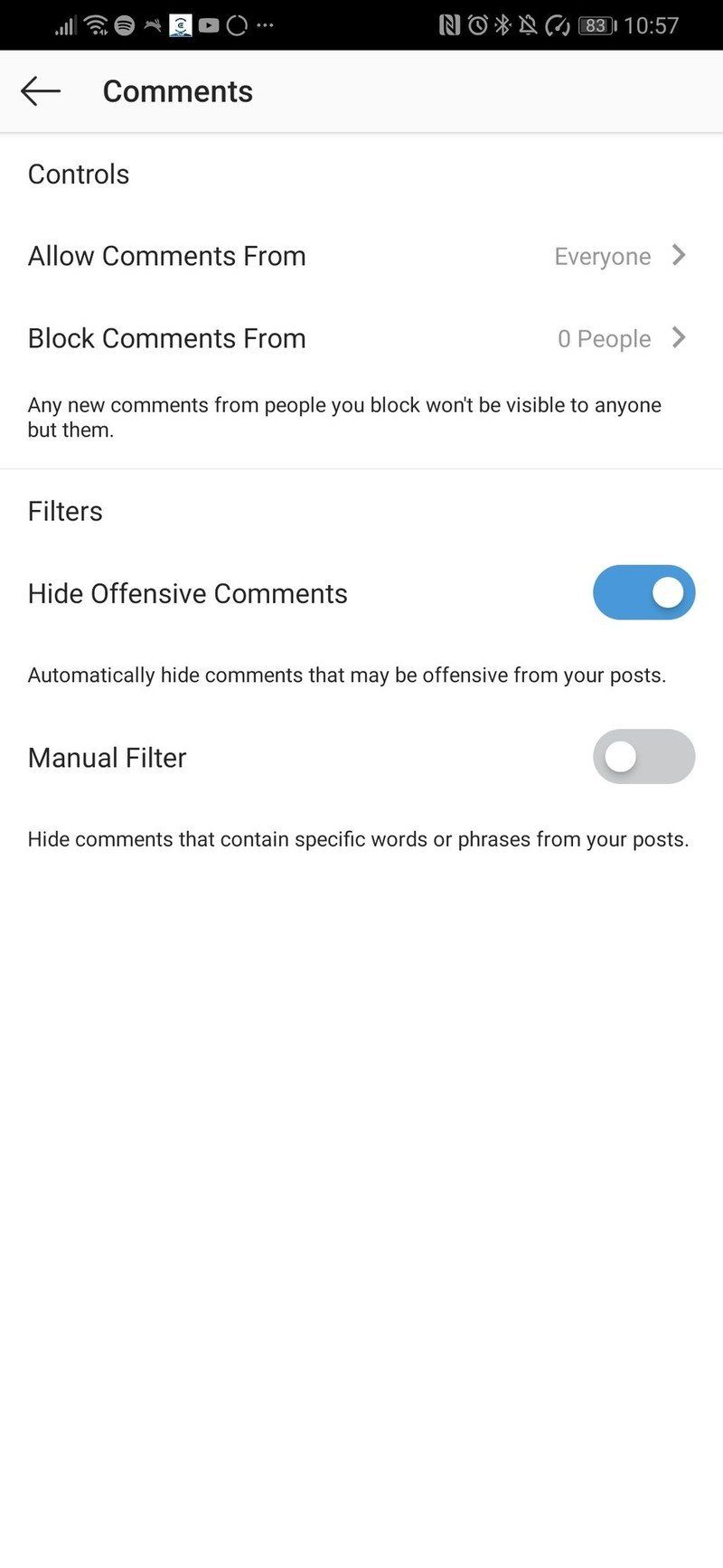This image appears to be a screenshot of a settings menu from a smartphone. The menu, likely belonging to a social media application or a website comments section, allows the user to modify who can comment on their posts. The background of the menu is white with black text for enhanced readability.

At the very top of the screenshot, there is a task bar, indicative of a mobile device interface. Beneath the task bar, the header reads "Comments", accompanied by a back arrow icon suggesting that users can navigate back to a previous menu.

The settings are divided into different sections. The first section is labeled "Allow comments from," and it is set to "Everyone," meaning any user can comment on the posts. Directly below, there's a section titled "Block comments from," with a note indicating "0 people" are currently blocked. A help text below this informs users that new comments from blocked individuals won't be visible to anyone but the comment's author.

Further down, there are toggle switches for comment filtering options. The first switch is labeled "Hide offensive comments," with the description "Automatically hide comments that may be offensive from your posts," and this option is turned on. The second switch is labeled "Manual filter," described as hiding comments that contain specific words or phrases, and this option is turned off.

In summary, the screenshot showcases a detailed comments management system within a mobile application, highlighting options for allowing, blocking, and filtering comments to maintain a positive user experience.